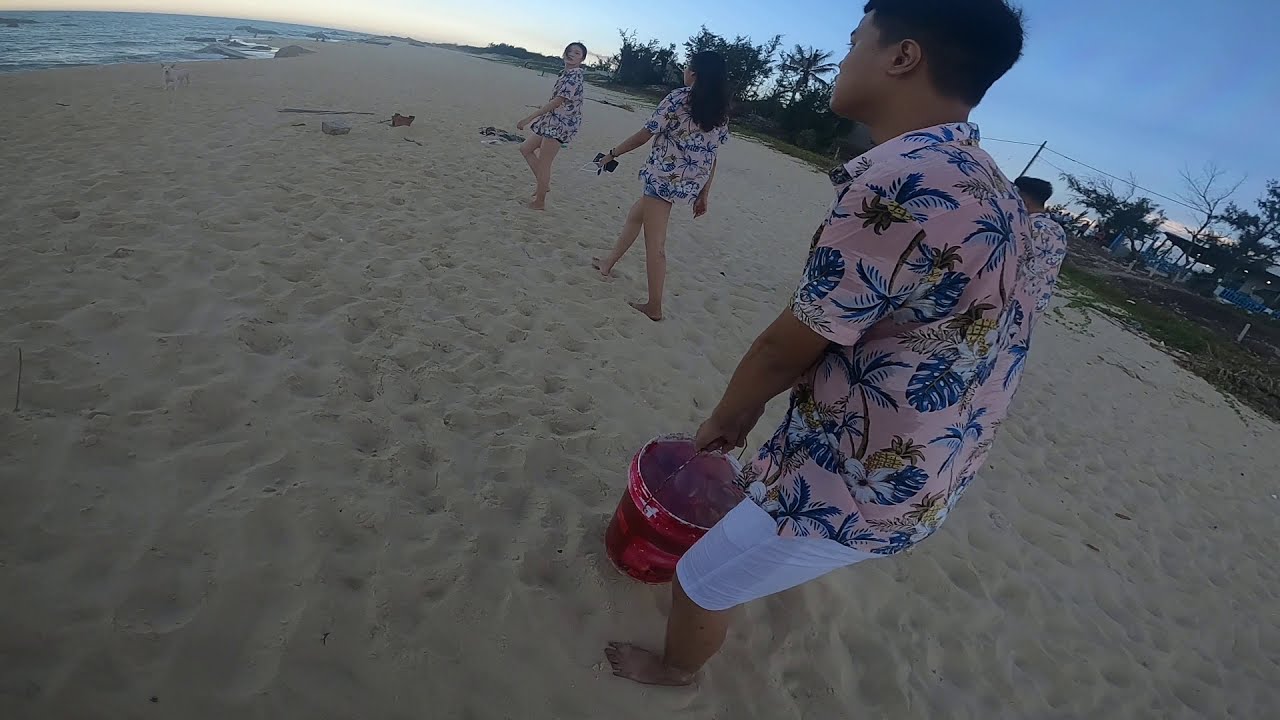The photograph captures a bright, almost dusk scene at the beach, where the sky transitions from blue in the top right corner to a white hue toward the left. Four individuals, two men and two women, all barefoot and dressed in identical pink, button-up shirts adorned with blue coconut trees and pineapples, walk on the sandy shore. The young man at the front, clad in white shorts, carries a red bucket likely filled with water. The sandy beach stretches towards the ocean visible in the upper left, while a strip of grass and small trees runs from the right side towards the left. In the background, the second man is partially visible, and the two women walk ahead, one appearing to converse with the other, who has long hair and holds a cell phone in her left hand. The serene beach setting is only interrupted by the distant grass and the calm ocean water, complementing the idyllic scene.